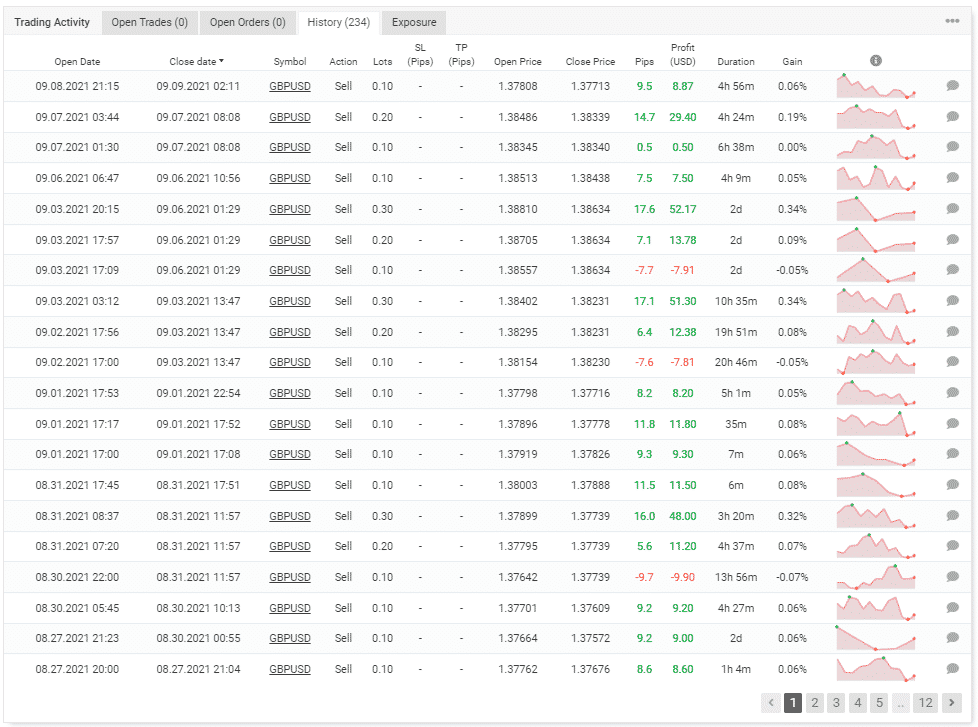A descriptive caption for the image could be:

"This image showcases a stock tracking webpage featuring a clean, white background with five tabs at the top labeled 'Trading Activity', 'Open Trade', 'Open Orders', 'History', and 'Exposure'. The 'History' tab is currently selected. The page displays a detailed table with approximately ten columns, each with headings such as 'Open Date', 'Close Date', 'Symbol', 'Action', 'Lots', 'SL Pips', 'TP Pips', 'Open Price', 'Close Price', 'Pips', 'Profit USD', 'Duration', 'Gain', and a column denoted by a gray circle with an 'i' in the center. This last column contains small charts depicting the rise and fall of stock values, illustrated by a thin pink line with a pink dot indicating the low point and a green dot marking the high point. The 'Open Date' column lists dates ranging from 09-08-2021 to 08-27-2021. At the bottom right corner of the page, there are several navigational boxes indicating a total of 12 pages of stock information."